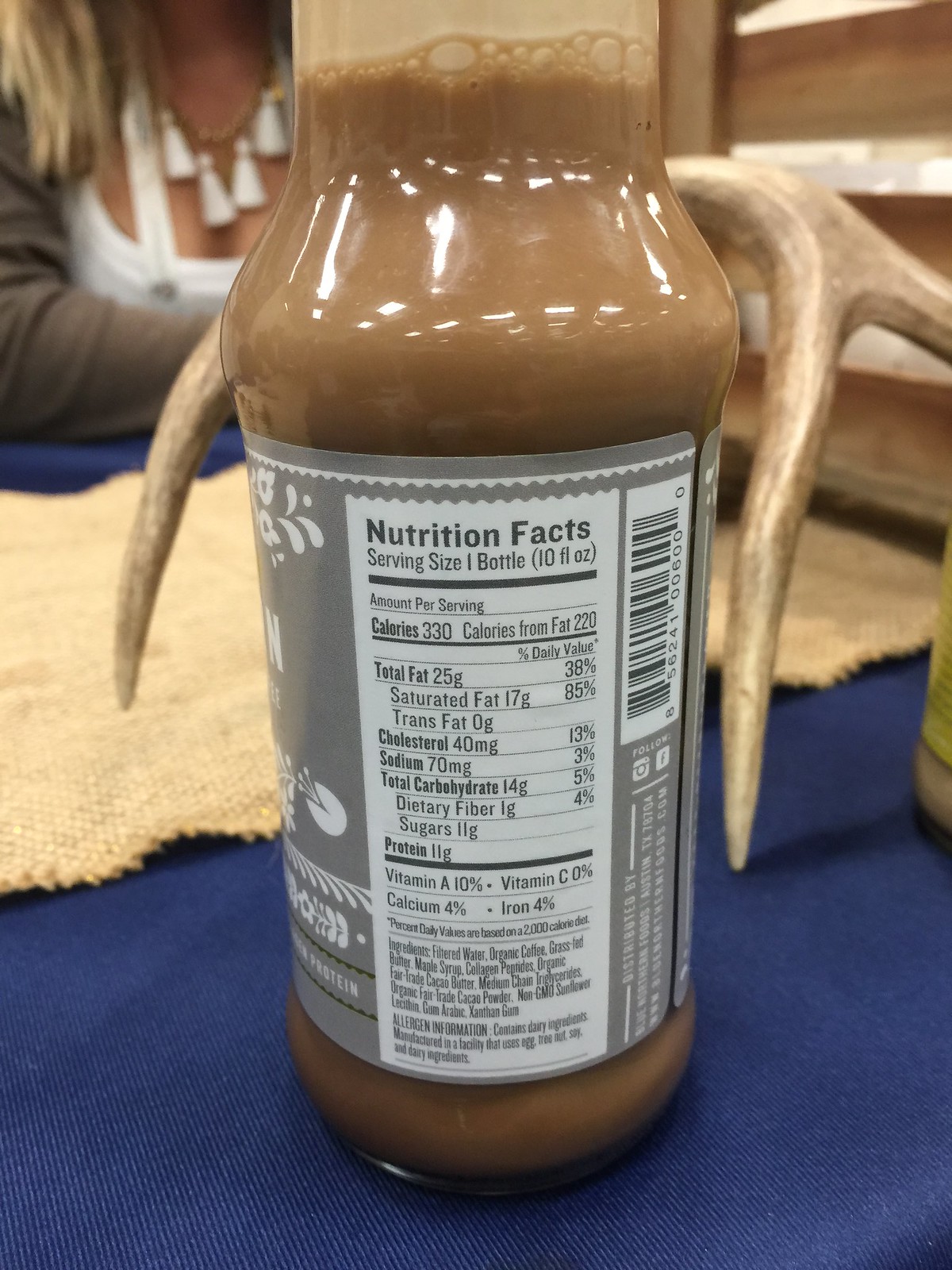A close-up photograph captures the Nutrition Facts label on the back of a bottle of what appears to be chocolate milk. The beverage is housed in either a plastic or glass bottle, with light reflecting off its top, suggesting the material's glossy nature. The bottle is positioned on a blue tablecloth, which adds a vibrant backdrop. In the background, a beige woven table runner extends across the table. Opposite the bottle, a woman is partially visible from the neck down. She has blonde hair and wears a necklace adorned with white tassel charms. Her attire includes a white shirt layered with a grey or brown sweater. The bottle's grey label clearly displays the nutritional content: a serving size of 1 bottle, 330 calories, 25 grams of fat, 40 milligrams of cholesterol, 70 milligrams of sodium, and 14 grams of carbohydrates. Additionally, a barcode and further text are present on the label, contributing to the information provided.